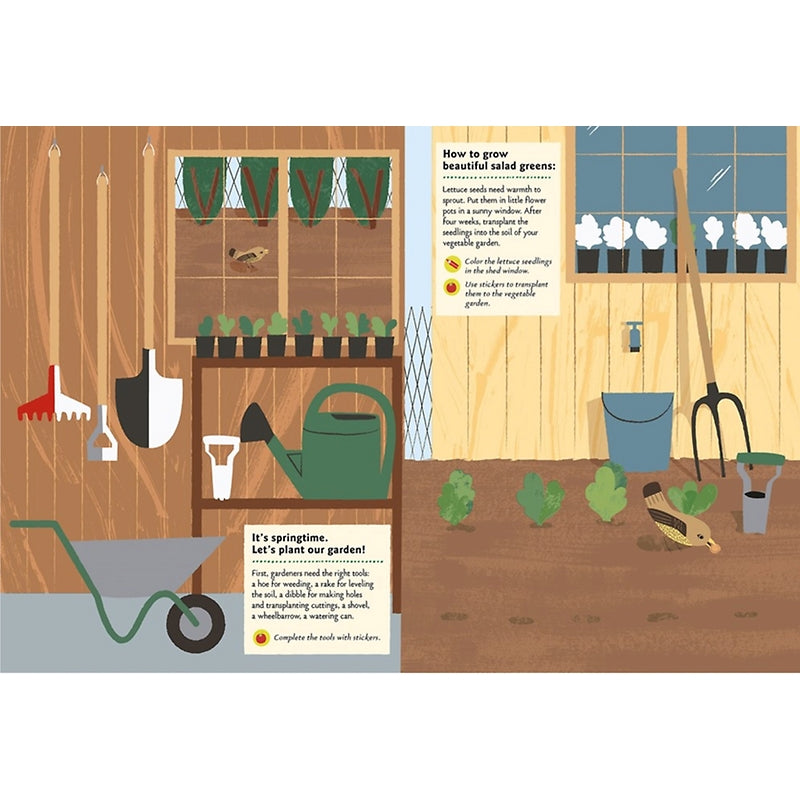This detailed illustration, approximately six inches wide by four inches high, is divided into a left and a right section, both depicting scenes related to gardening. 

On the left side, we see the interior of a shed meticulously organized with essential gardening tools. The gray floor supports wooden walls adorned with a window, through which bushes and a bird are visible. Below the window, a shelf holds potted plants, while a second shelf displays a green watering can and a white planter. Hanging on the left wall are a shovel, hoe, and rake, with a wheelbarrow positioned at the bottom. A prominent light-colored square with black print reads, "It's springtime, let's plant our garden," followed by a detailed paragraph about gathering the right tools: a hoe for weeding, a rake for leveling the soil, a dibble for making holes, a shovel, a wheelbarrow, and a watering can.

The right side transitions to an outdoor scene. The ground is brown dirt, interspersed with small green plants and a bird pecking at seeds. The shed's exterior is made of light brown wood, featuring the same window with visible potted plants. Below the window, a pitchfork and a bucket sit under a water spigot. A white rectangle on the shed bears the heading, "How to Grow Beautiful Salad Greens," with detailed instructions for planting lettuce: starting seedlings in flower pots on a sunny window and transplanting them into the garden after four weeks. This side captures the essence of the growing process, reinforcing the theme of spring gardening.

Overall, the illustration serves as an educative and engaging guide for budding gardeners, blending indoor preparation with outdoor planting practices.